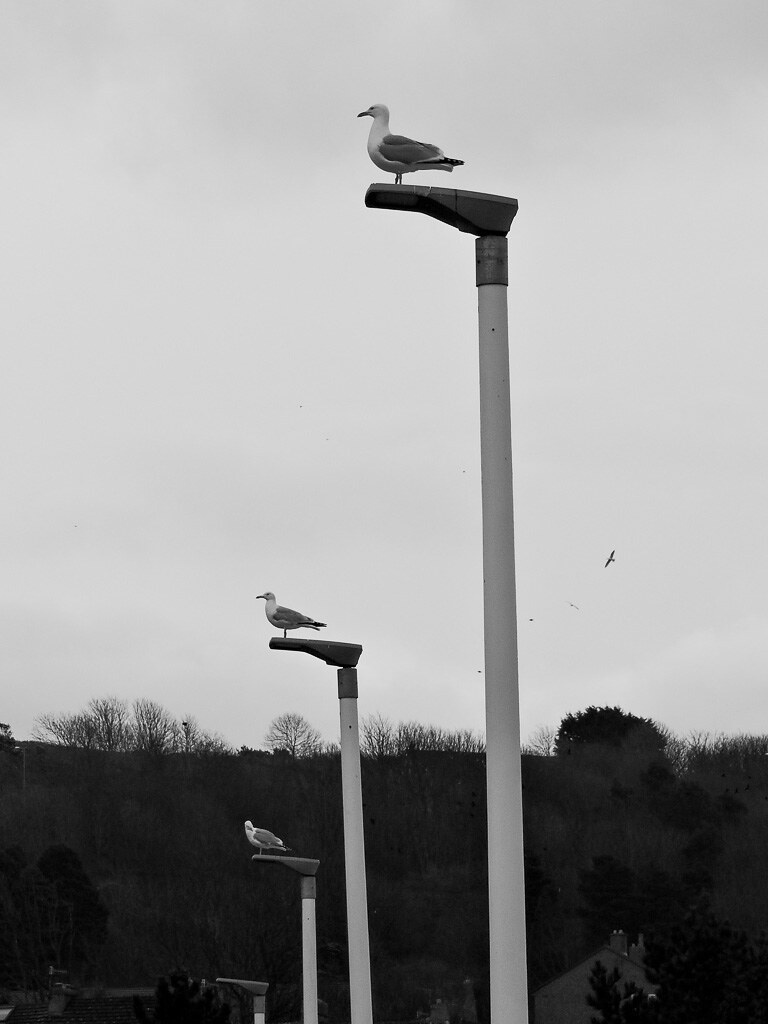This black and white photograph captures an artistic outdoor scene, dominated by four tall street lamps stretching upwards into a cloudy sky. Arranged in a receding angle from right to left, the tallest lamp post stands right of center, while the other three lamps decrease progressively in height. Perched atop these lamps are seagulls, each facing towards the left. The rightmost three seagulls sit serenely, with the leftmost one preening its feathers. High above, a group of four birds soars in the sky, adding depth to the composition. The horizon line, located in the bottom third of the image, features the silhouette of trees and rooftops, casting shadowy figures against a sheet of gray sky. The photograph's grayscale tones enhance the moody, serene atmosphere of this everyday yet evocative scene.